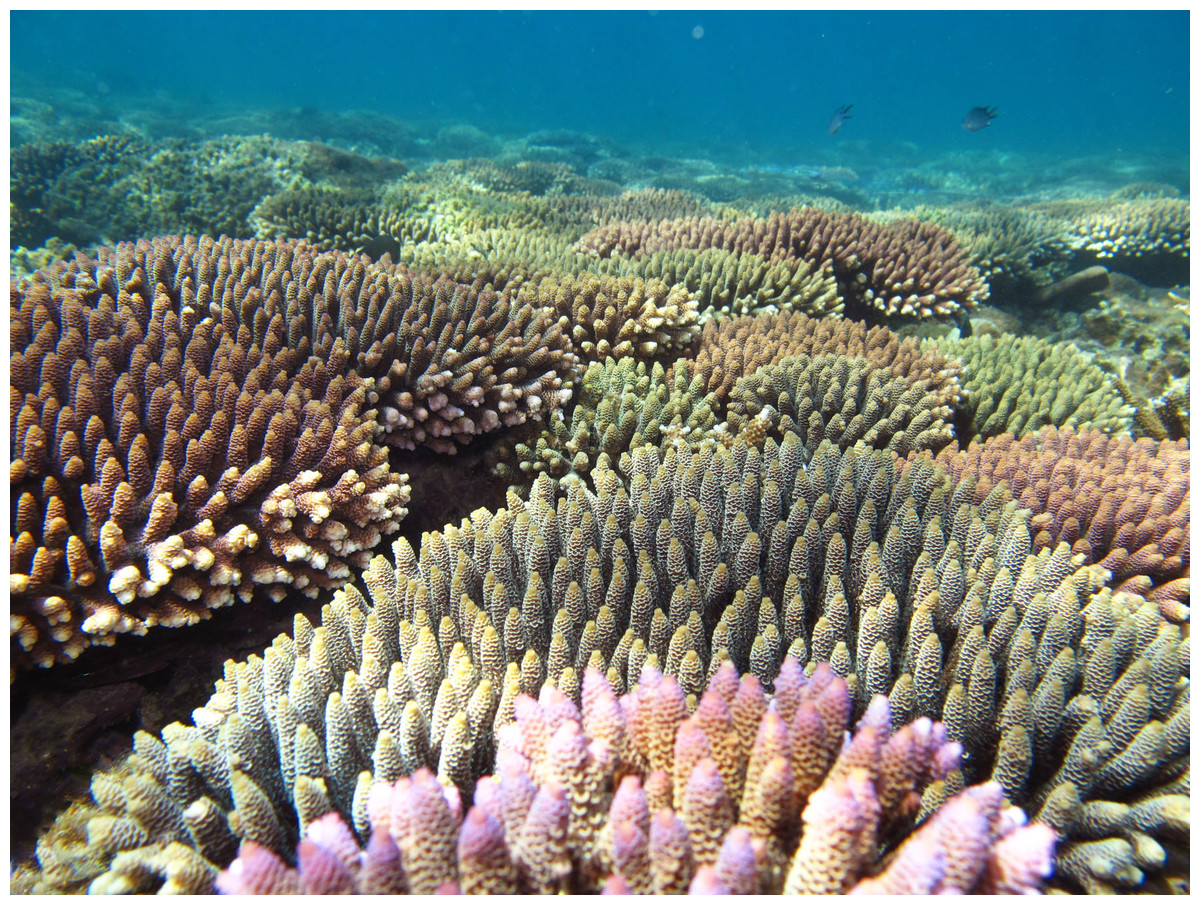This photograph captures an underwater scene on the ocean floor, blanketed with an array of vividly colored corals. The corals, resembling small bushes with numerous finger-like protrusions, stretch across the seafloor and display a spectrum of colors, including lavender, green, rust, pink, gray-green, and brownish-pink. In the foreground, there is a close-up of corals featuring distinct hues of green and light yellow, with the various colors blending seamlessly as they extend into the background. The point of view is nearly at the level of the coral, just slightly elevated, adding depth to the image. On the right side of the background, two flat fish swim gracefully, illuminated by the scattered, subtle sunlight that filters through the water, suggesting the scene is relatively shallow. The entire underwater landscape is bathed in this soft light, enhancing the visibility and detail of the vibrant coral bed.